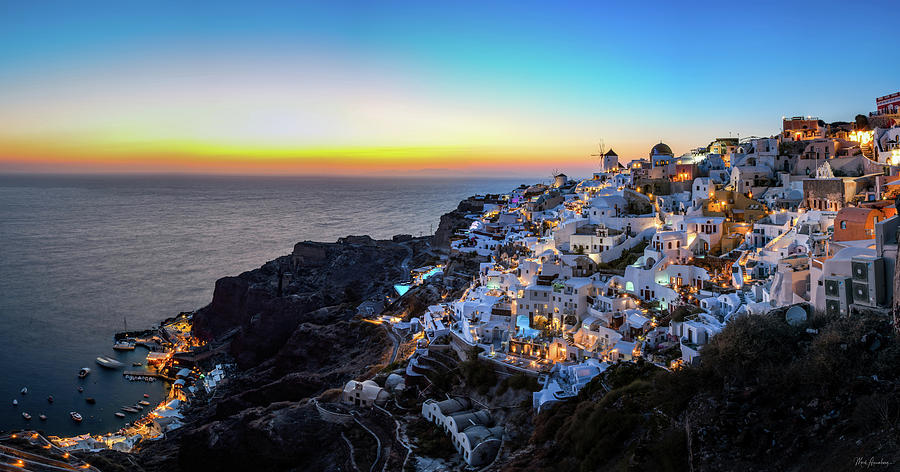This color photograph captures a stunning, overhead view of a village built along a cliffside overlooking a calm, blue ocean. The village, reminiscent of a typical Greek town, is composed of numerous white houses clustered together on the right side of the image, built up the dark cliffs. The tranquil water on the left side of the image reflects the deep blue of the darkening sky, with a glowing orange sunset in the background casting a warm light over the scene. At the base of the cliffs on the lower left, lights illuminate what appears to be a dock or waterfront area, where several boats are moored. Additionally, you can make out some trees and shrubs growing amidst the rocky landscape, adding a touch of greenery to the picturesque scene. The combination of twinkling house lights, serene waters, and vibrant sunset creates a beautifully composed and atmospheric photograph.